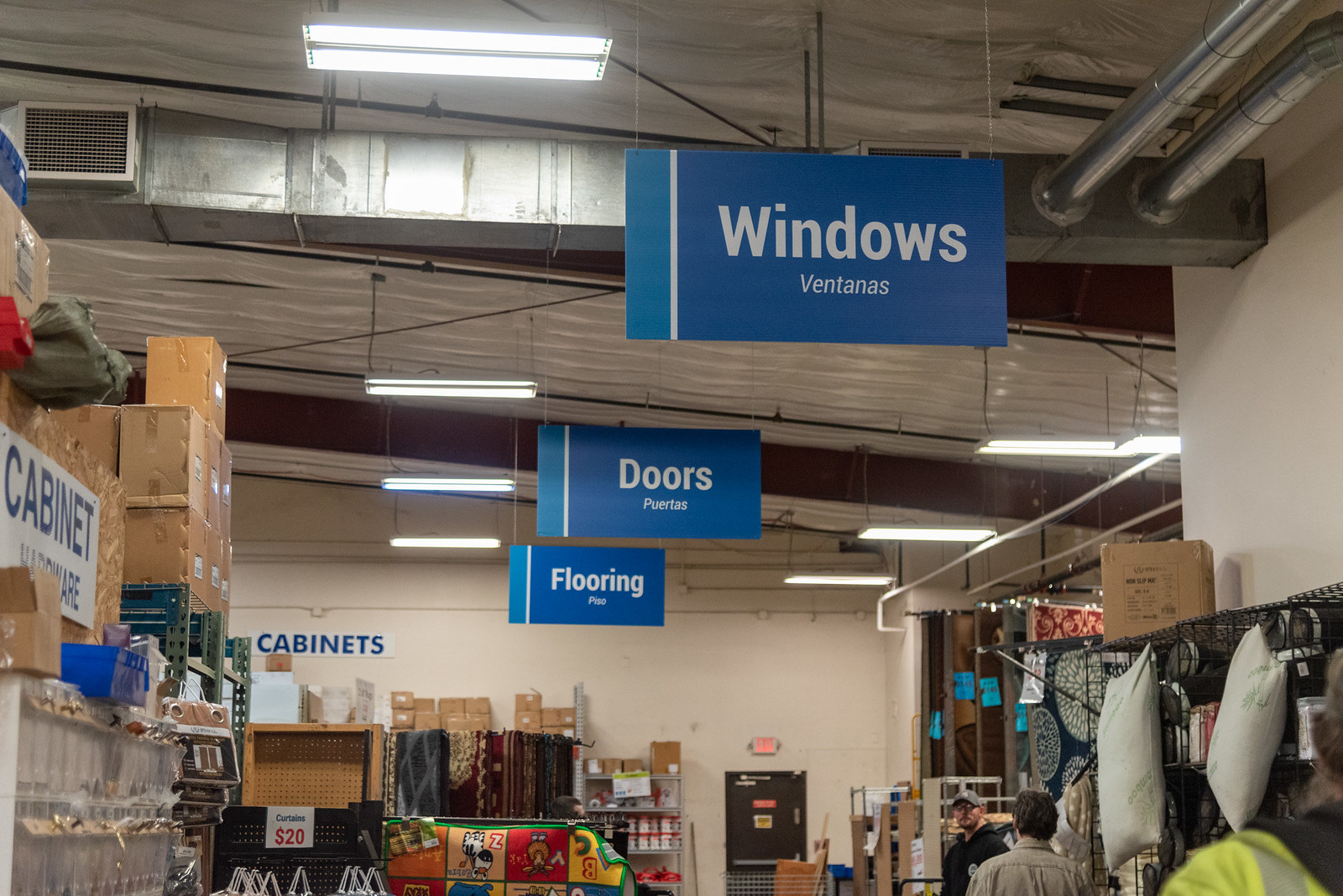This photograph captures the interior of a home improvement store from a raised perspective, likely taken with the camera held above the photographer's head. The image prominently features an unfinished ceiling, exposing ductwork, insulation, and hanging light fixtures. 

Dominating the upper half of the image are various aisle markers in blue, clearly labeled in both English and Spanish. These markers identify different sections such as "Windows/Ventanas," "Doors/Puertas," and "Flooring/Piso." 

On the left side of the image, a sign indicates the "Cabinet Hardware" section, featuring numerous compartments for various hardware pieces. In the background, a wall with the word "Cabinets" suggests different cabinetry options available in the store.

To the right, a display wall showcases an assortment of pillows and decorative items. Further in the distance, an exit sign is visible above a back door, contributing to the utilitarian and rustic ambiance of the store.